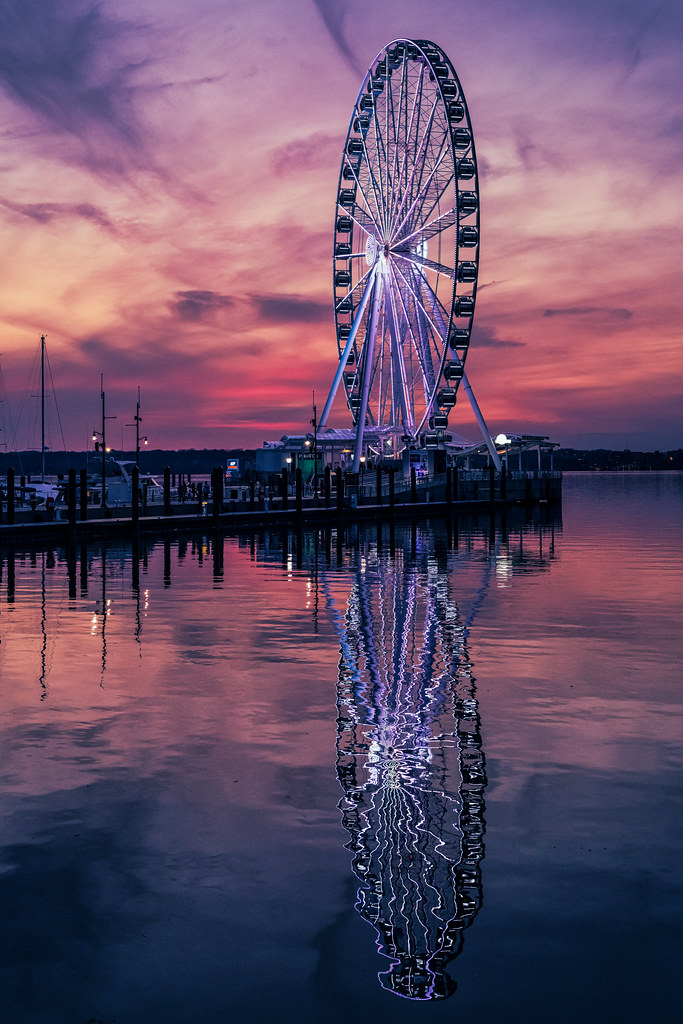The image captures an enchanting evening scene featuring the Capitol Wheel on a wooden pier at National Harbor, Washington, D.C. The sky is a canvas of vibrant sunset hues, with purples, pinks, and deep reds blending together, creating a stunning backdrop. The ferris wheel, positioned centrally in the image, is illuminated and casts a striking reflection on the glassy, calm waters below, albeit with an odd angle that seems a bit surreal. Surrounding the pier are various small boats and yachts docked nearby, as well as buildings likely for rentals. The pier itself is adorned with lights, enhancing its picturesque quality. In the background, across the water, is the distant coast, adding depth to the composition. This well-lit ferris wheel, with its numerous seats or "cars," stands prominently, making the overall scene both mesmerizing and dynamic.